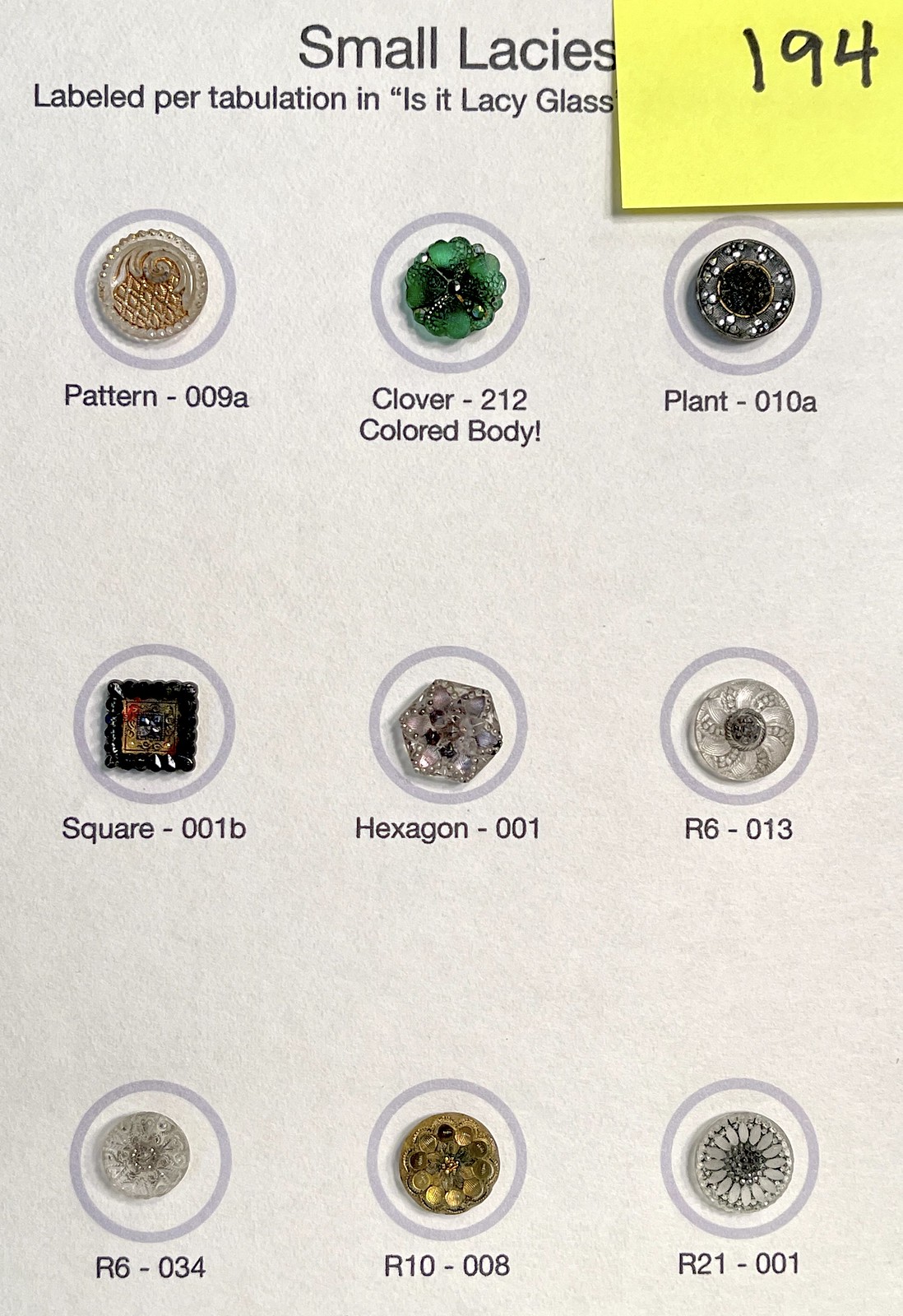This image depicts a light gray piece of paper labeled at the top with dark gray text reading "Small Lacies." Below this heading, it says "labeled protabulation" and a partially covered phrase referencing "Lacy glass." A yellow sticky note with the number "194" in black print is affixed to the upper right corner. The paper features a 3x3 grid of gray circles, each containing a unique, shiny object centrally positioned within the circle. 

In the top row, from left to right, the circles contain different objects: the first is a round, brown and clear object labeled "Pattern 009-A"; the second is a round, green glass-looking object labeled "Clover 212 Colored Body"; and the third is a black and white shiny circle labeled "Plant 010-A." The subsequent two rows include a mix of round, square, and hexagon-shaped objects, each clearly centered in its respective circle with their identifiers placed beneath them. Specifically, some of the labels featured in these rows include "Square-001B," "Hexagon-001," "R6-0013," "R6-034," "R10-008," and "R21-001."